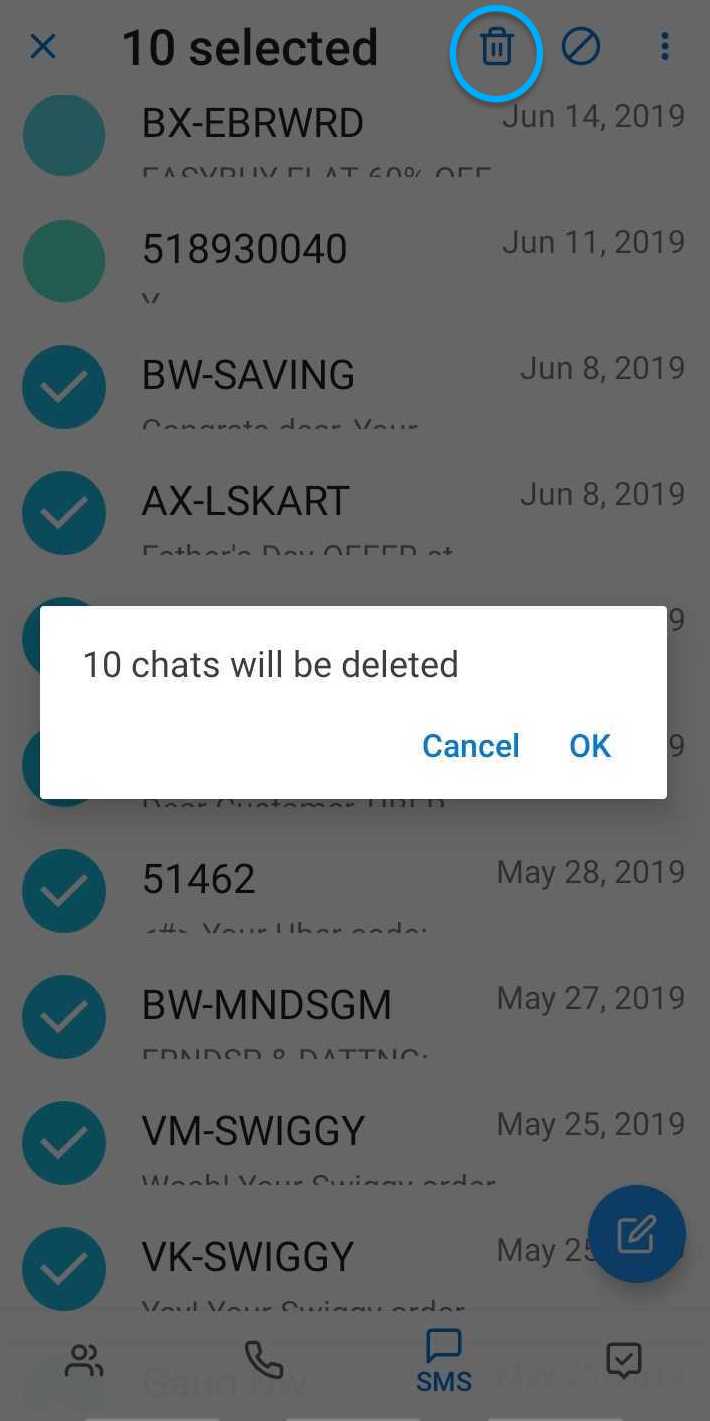The image portrays a smartphone screen in portrait mode, dimly lit to emphasize an overlaying box. This box prominently displays options for managing chat conversations. In the top left corner, a small blue "X" is visible. To the right, bold black text announces "10 selected." The top-right corner features three icons: a trash can encircled in light blue, a prohibited sign, and three vertical dots.

Vertically aligned on the left side of the box are a series of circles, alternating between blue and green. The upper two circles are empty, while the remaining ones contain white check marks. Adjacent to these circles, strings of black alphanumeric text are displayed, such as "PX-EBR WRD," each accompanied by a date like "June 14, 2019."

In the center, a white rectangular notification with black text declares "10 chats will be deleted," referring to the check-marked items. Below this message, two buttons—"Cancel" and "OK"—both in blue, offer action choices. 

Further down, a blue circle icon with a pen and paper is present, potentially for composing new messages. At the very bottom of the screen, there is a navigation bar with icons representing contacts, a phone, and "SNS," the latter highlighted in blue and featuring a small box with a checkmark.